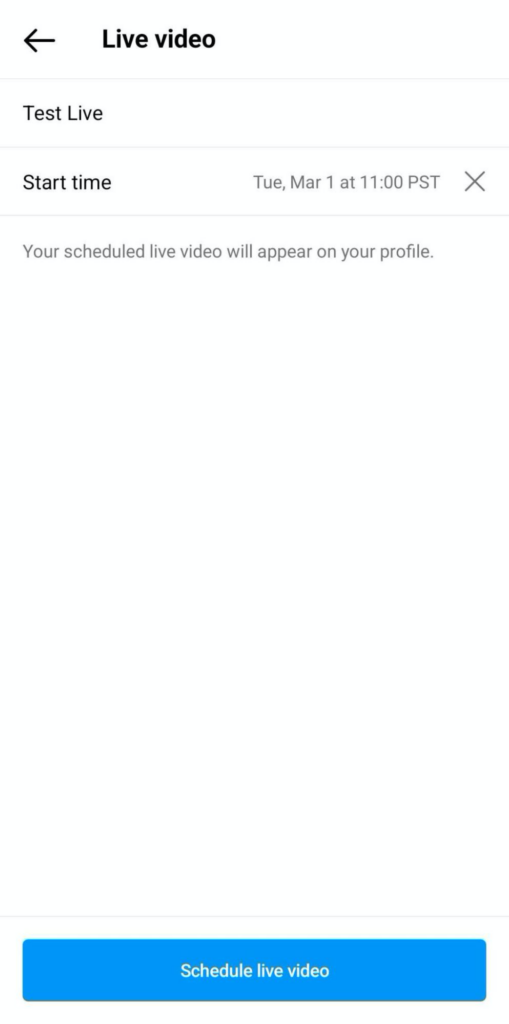The image displays a smartphone screen showcasing a user interface for scheduling a live video. At the top left, there's a label "Live Video Test" with the scheduled start time set for Tuesday, March 1st, at 11:00 AM PST. Below this, the interface informs the user that their scheduled live video will be visible on their profile once it's set. A prominent blue rectangle button is present, labeled "Schedule a Live Video." The background includes a subtle left arrow icon, reinforcing the context of navigating through the app's scheduling feature. The text is consistently clear, although some details, such as the reminder that the live video will appear on the profile, are in a smaller font size.